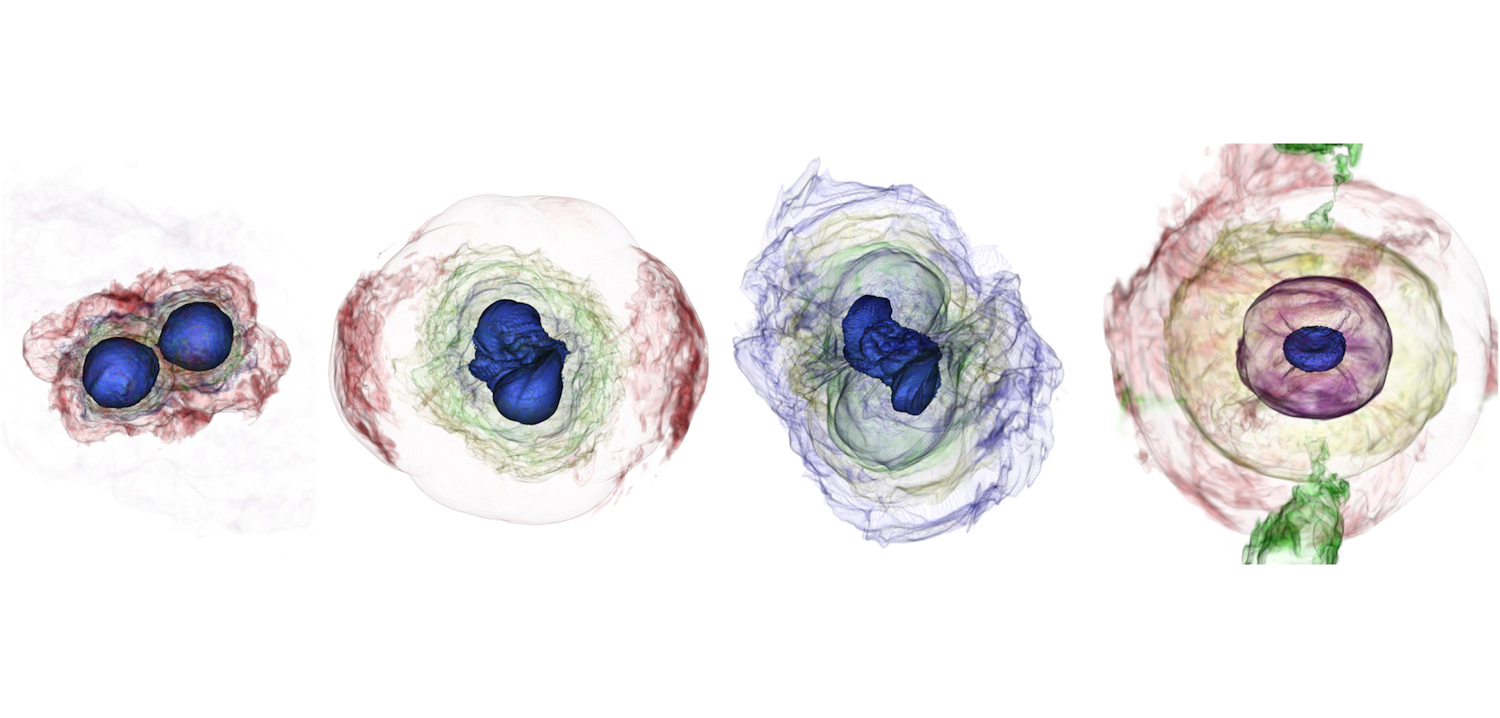The image consists of four distinct illustrations, each featuring a central blue circular or oval-shaped object, reminiscent of either blueberries or nuclei, set against various colored surroundings. The first illustration on the far left shows two blue circles nested within a blend of orange, green, and wavy colors, creating a vibrant, almost biological or abstract art effect. The second illustration features a prominent blue mass at its center, encircled by green squiggly lines and surrounded by a mix of pink, white, and muted pastel hues. This might represent a larger singular entity or a different stage of the central object's evolution. The third illustration presents another central blue blotch, somewhat altered in configuration from the previous image, within a mix of green and blue elements, possibly signifying a continuation in form or a different state. The fourth and final illustration portrays a single blue central figure surrounded by intricate patterns of pink, red, and green, potentially hinting at an artistic depiction of an eye, complete with a blue ‘pupil’ and a reddish ‘iris’. The abstract and detailed renderings create an enigmatic and visually engaging series, suggesting interpretations ranging from biological cells to stylized representations of eyes or fruits.